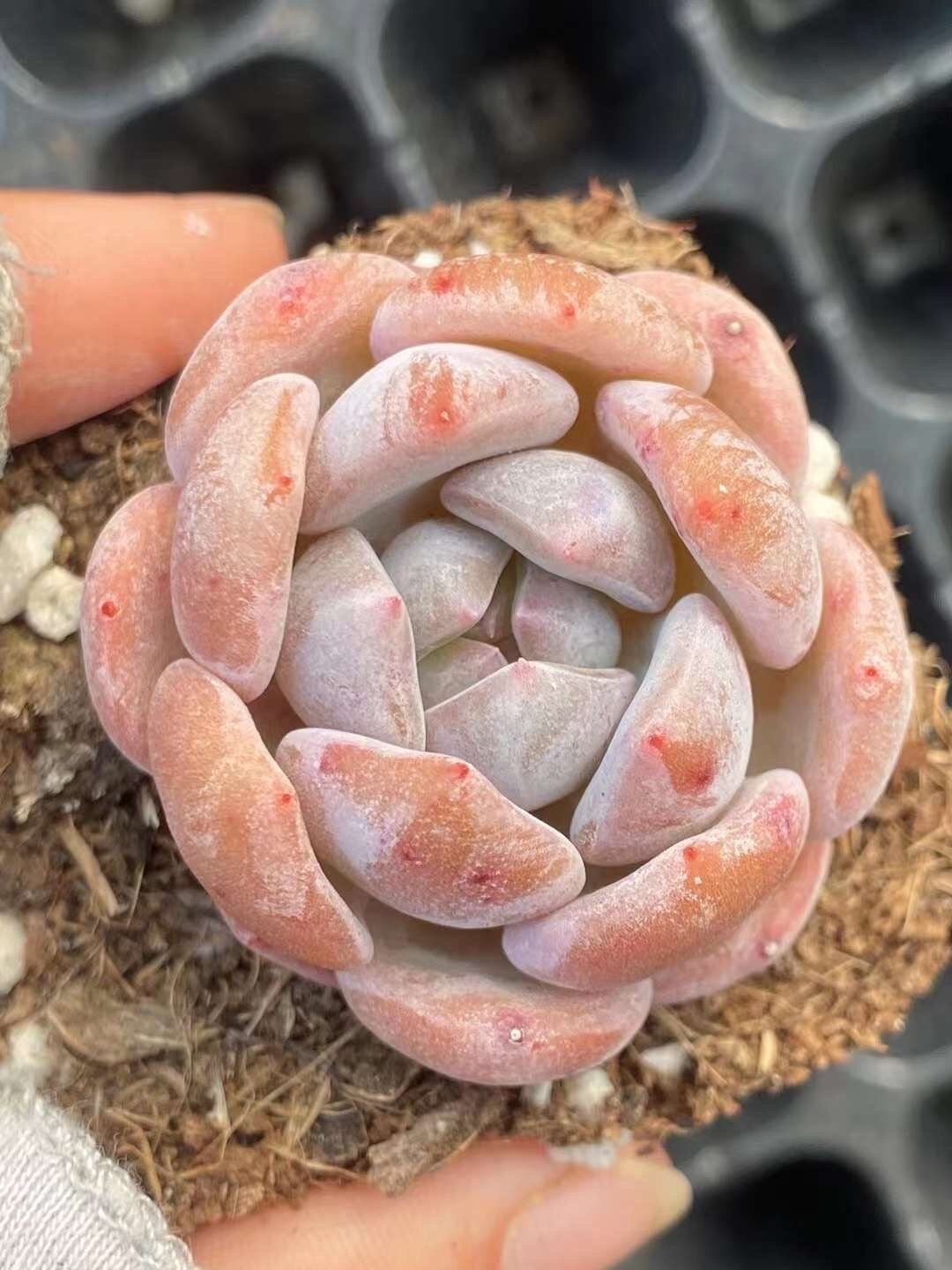The image depicts a close-up view of a pink and grey succulent plant, resembling a cluster of bulbous, peachy petals covered in a frosty, powder-like substance. The plant forms a circular, bouquet-like shape, with its diameter estimated to be around three to four inches. A person, likely female based on the appearance of her long thumbnail, is delicately holding the plant by its soil-covered base with her thumb and forefinger. The vibrant succulent appears to be freshly lifted from a compartmentalized black tray visible beneath, suggesting it is part of a collection or arrangement of similar small, flowering cactus-type plants. The scene is set against a backdrop of dirt and dead vegetation, adding a naturalistic touch to the photograph.